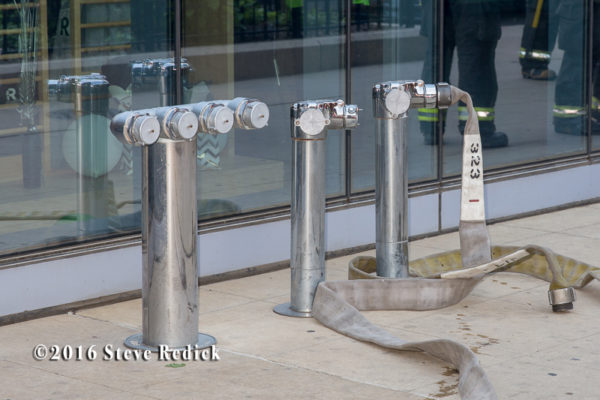In front of a glass wall, likely part of a commercial building or fire department, three silver fireman posts are positioned on a beige-tiled floor. The leftmost post features four round nozzles on top, with a silver circular pole beneath them. The middle post is thinner and has two nozzles. Notably, both of these posts have meters, which may serve as connectors. The rightmost post is identical to the middle one but includes a grey hose attached to its opening. The hose, marked with the number 323, appears to be empty and winds around on the floor, connected to the post. In the background, large reflective windows show what seem to be firemen wearing pants with reflective bands. The colors visible in the image include brown, silver, gray, tan, white, black, red, green, and yellow. Notably, the image contains the text "2016 Steve Reddick" at the bottom left.